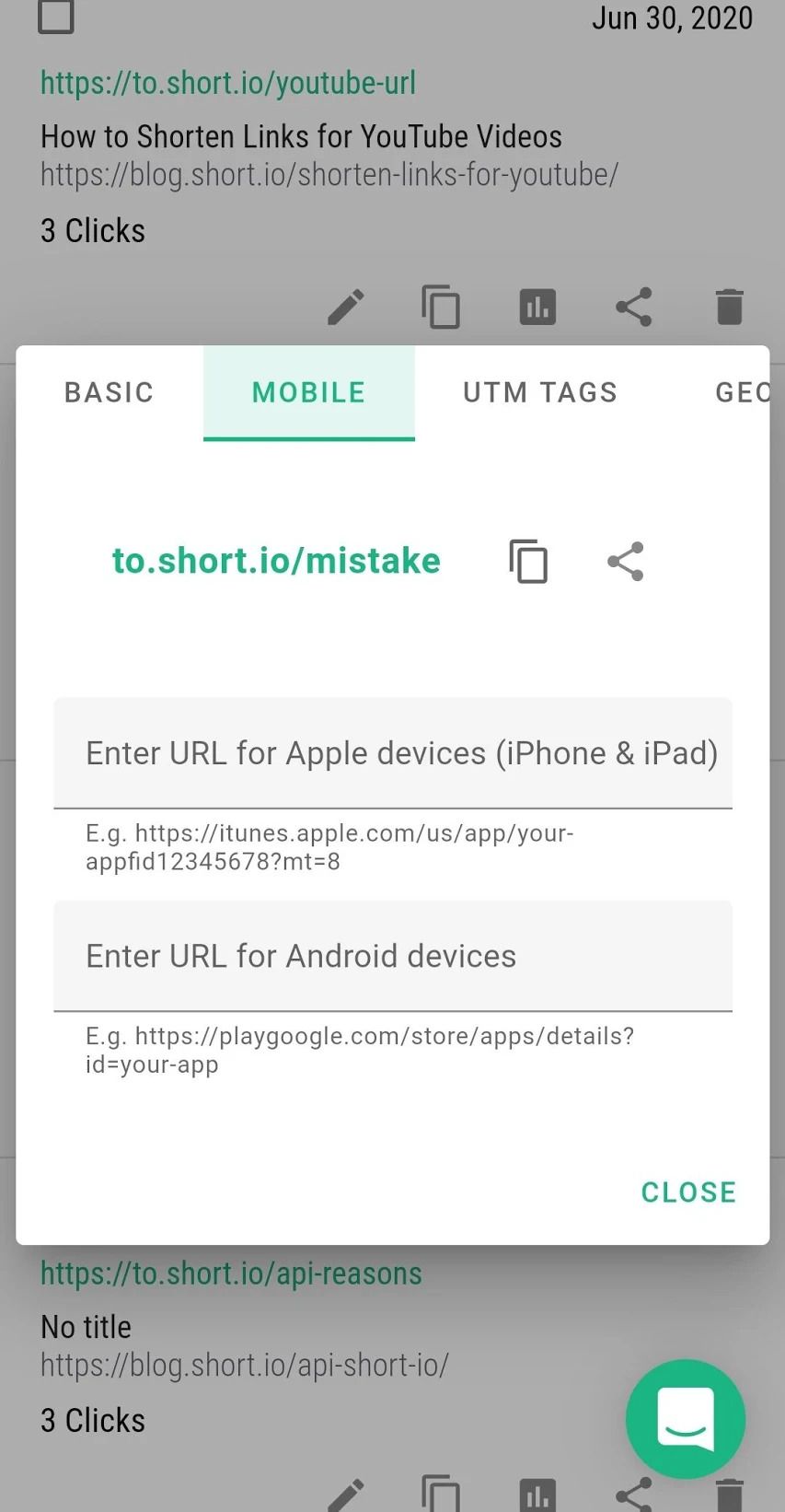The image depicts a smartphone screen displaying a partially obscured app interface due to a pop-up window. The background is grayed out and shows the date "June 30th, 2020" along with a URL: "https://short.io/YouTube.url" highlighted in green. Below the URL, the text reads "How to shorten links for your YouTube videos," followed by another URL, and then the phrase "three clicks." At the bottom, there are several icons including a pencil, two overlapping three-dimensional squares, a graph-like icon with three dots connected by lines, and a trash can symbol.

The pop-up window prominently features the title "Basic Mobile UTM Tags," with "Mobile" selected and highlighted in green. Another green URL is displayed: "https://to.short.io/mistake". The pop-up includes options to input URLs, specifically marked sections for "Apple devices (iPhone and iPad)" and "Android devices." Each input field offers example URLs for guidance. The same icons from the background—two overlapping 3D squares and a graph-like icon with three connected dots—reappear within the pop-up for further navigation or action.